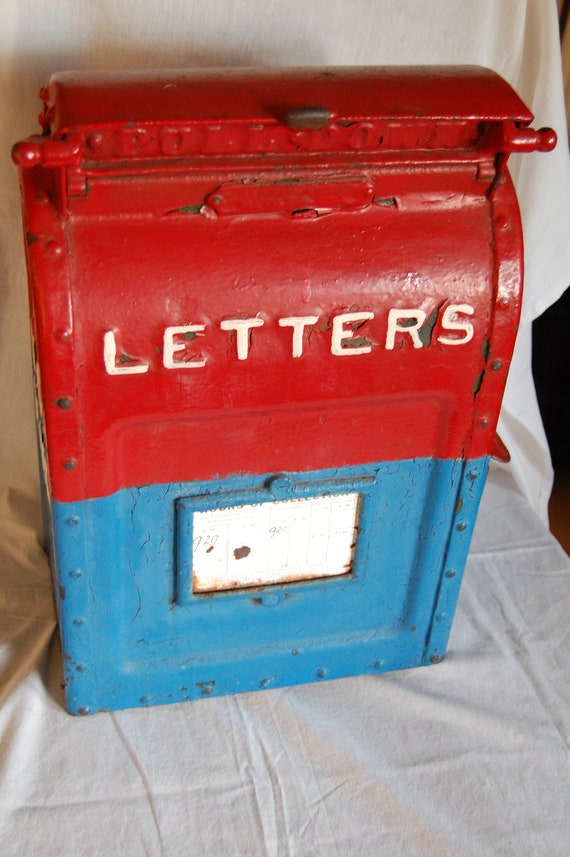This is a detailed color photo of an antique, metal mailbox, which appears to be photographed indoors, resting on a white cloth that covers a table. The mailbox has a distinctive vintage look, with chipped and cracked paint indicating its age. The top portion of the mailbox is painted red, featuring the word "letters" prominently in white letters. The top is rounded and includes two small handles on each side of this red section, marked with "pull down," suggesting they are used to open the mailbox. From the midpoint down, the mailbox is painted a medium blue. On this blue section, there is a small rectangular panel with a white center that appears to display a faded schedule or collection times, with "920" faintly visible. The general appearance of the mailbox evokes a bygone era, suggesting it was once mounted on the side of a building.